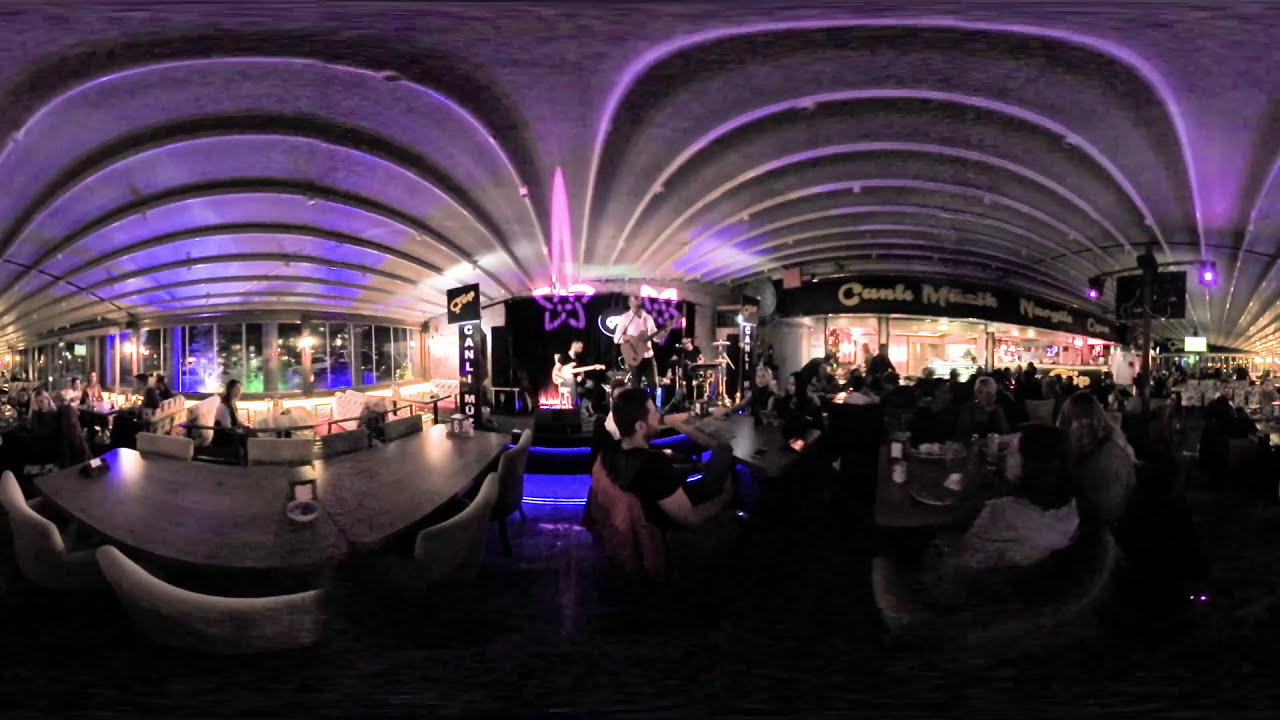In this detailed image of a restaurant that doubles as a nightclub, the scene is set with an array of vibrant colors from blue, purple, and green, cast by various lights. The interior boasts a distinctive scalloped ceiling, painted or lit to appear extensively purple. The ceiling features a series of arches on both the left and right sides, enhancing the architectural flair of the space. Accommodations include a variety of tables and chairs where patrons are seated, notably a prominent semicircular table on the left side, surrounded by cushioned, arch-shaped chairs which remain unoccupied. Throughout the room, additional tables host groups of diners, with the left side sparsely populated and the right side more crowded, highlighted by well-lit, mirrored glass windows.

Amidst the dining area stands a stage, illuminated by purple lights reflecting off the ceiling. A band is in full swing, featuring a standing guitarist, a seated guitarist behind him, and another musician on the right, somewhat obscured. The right side of the room is particularly notable for its glass windows that allow a view of the outside night, adding a luminescent glow to the darkly lit venue. Above one section of the restaurant, possibly near the glass area, a sign partially reads "CANL" followed by other indistinct letters, suggesting the name or theme of this chic, vibrant location.